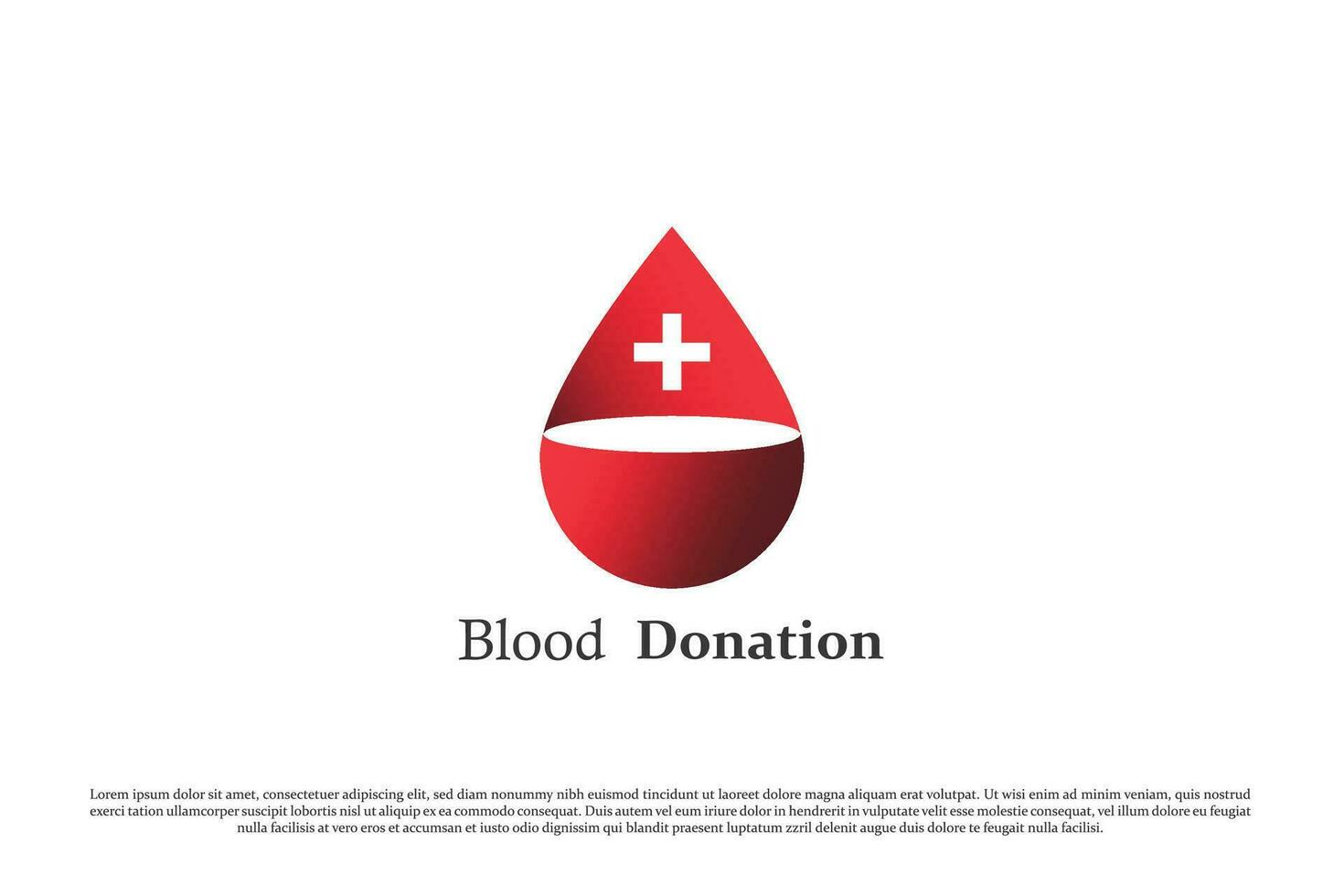This image features a stylized illustration of a blood drop, transitioning from a lighter red at the top to a darker red at the bottom, evoking a teardrop shape. Prominently situated in the upper portion of the drop is a white cross, while a white oval occupies the central area. Below the blood drop, the words "Blood Donation" are displayed in black text, with "Donation" emphasized in a bold font. Further below, three lines of placeholder text, resembling Latin ("Lorem ipsum dolor sit amet, consecetur, adipisci elit, sed do eiusmod"), stretch wider than the main image elements, adding to the design's visual depth. The entire composition is clean and devoid of additional backgrounds, borders, or people, focusing solely on the theme of blood donation.